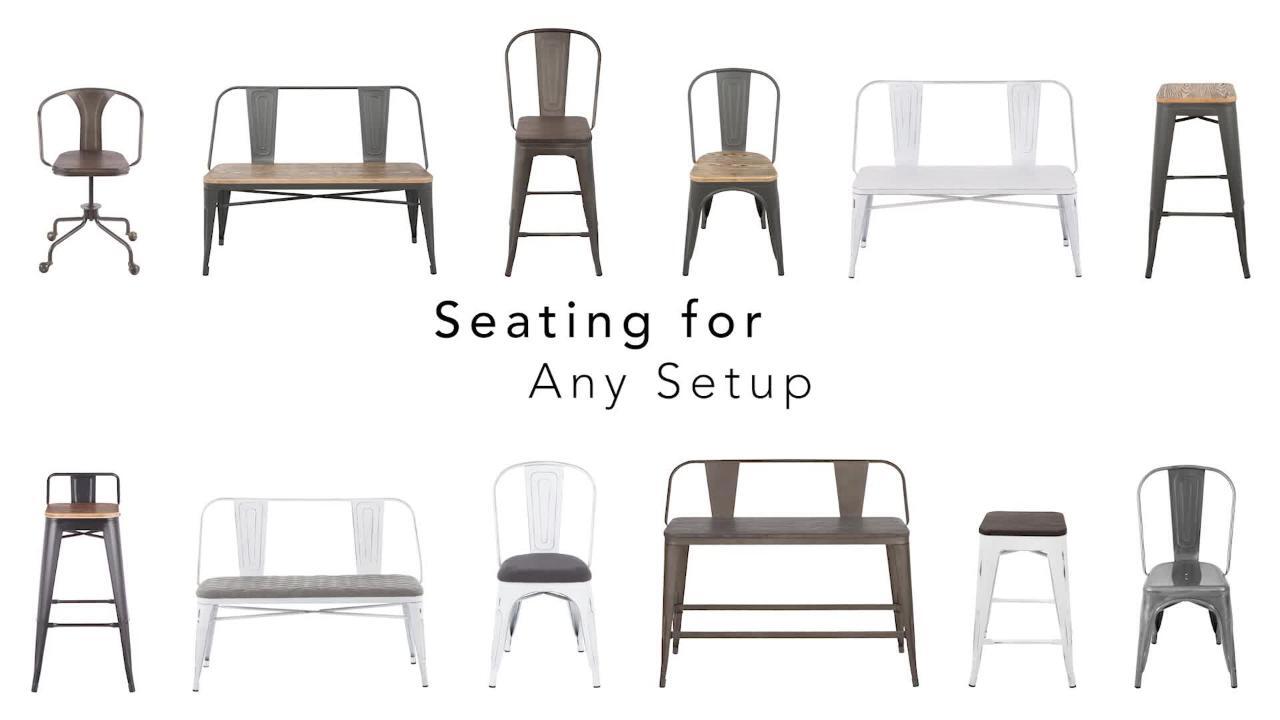This image, likely an advertisement for a furniture store, showcases a variety of seating options against a minimalist white background. The layout is divided into two horizontal rows, each featuring six different types of seating. The rows include a mix of office chairs, benches, bar stools, and dining chairs, crafted from metal and wood. Predominantly in shades of brown, beige, gray, and white, these seats are designed with a contemporary minimalist aesthetic.

In the top row, from left to right: a rolling office chair with a brown wooden back and seat, a slender two-person bench, a tall bar stool, a standard chair, a white-painted metal bench with a gray seat, and a traditional bar stool. The bottom row mirrors this arrangement with slight variations: a bar stool with a short back, a white bench with a medium-sized back, a white chair with a gray cushion, a taller brown bench with a short back, a backless white stool with a gray cushion, and a brown metal chair with no arms but a medium-sized back. The phrase "Seating for any setup" is positioned centrally between the two rows in brown lettering, reinforcing the theme of versatile seating arrangements for various needs.